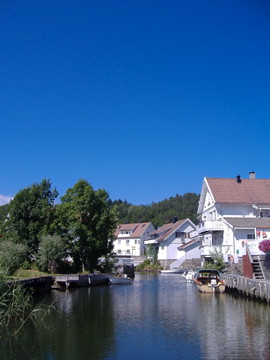This vibrant image captures a picturesque lakeside scene, likely in a European country such as France, Germany, or Switzerland. Dominating the right side of the image are three multi-storied white houses, possibly hotels, with chimneys and distinctive pinkish-reddish roofs, which might feature high steps to prevent flooding. To the left, verdant trees line the clear, still water, with boats, including a small green-topped fishing vessel, docked at a modest pier. The serene lake, with its mix of brownish-blue hues, reflects the lush, rolling hills and an azure sky, suggesting a warm, sunny day in spring or summer. The tranquil, idyllic backdrop of dense greenery and gently sloping hills enhances the charm of this apparent tourist destination.